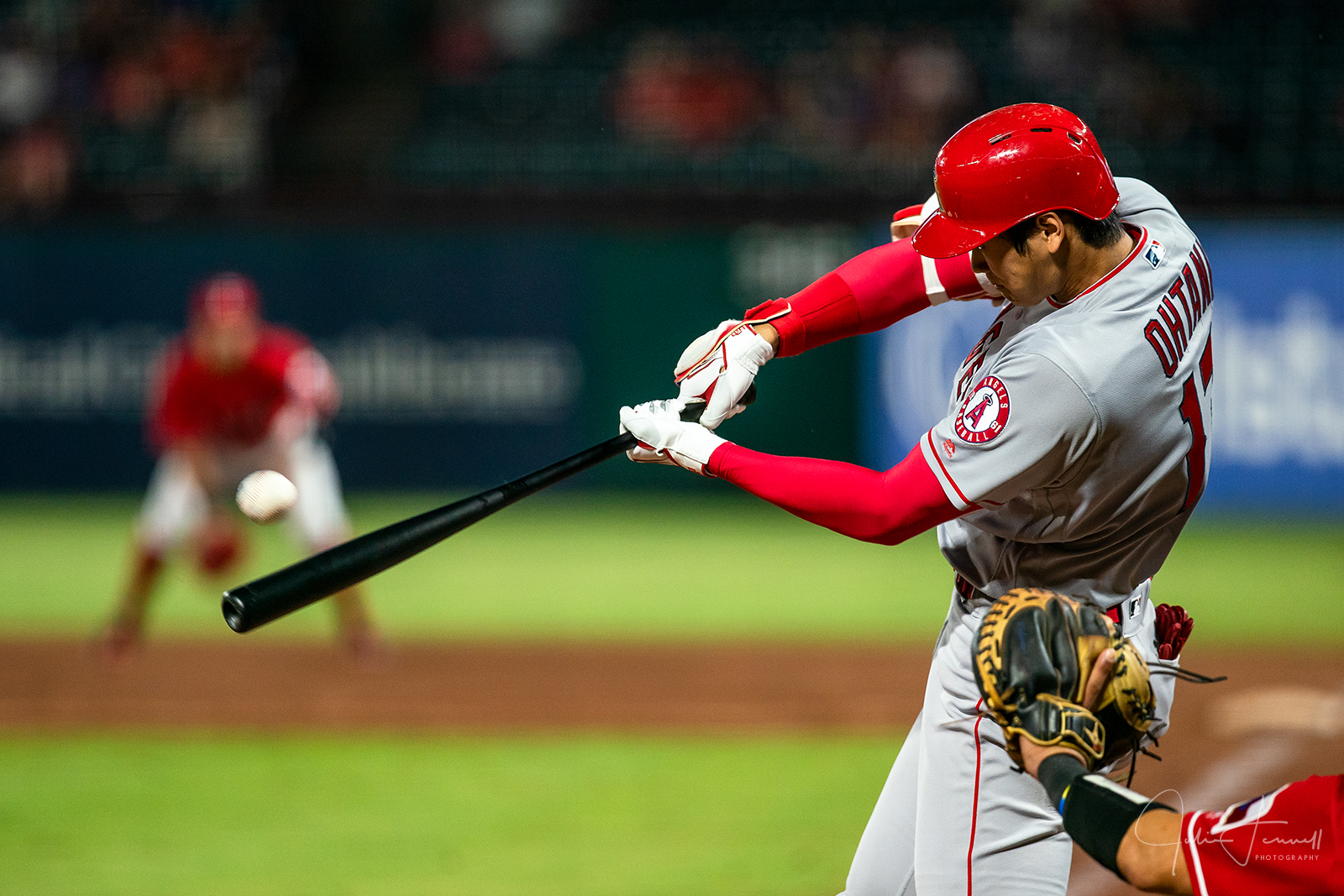The image captures a precise moment during a Major League Baseball game, featuring Shohei Ohtani of the Los Angeles Angels at bat. Ohtani, clad in a gray and red uniform with red sleeves, white gloves, and a red helmet, is swinging a black bat at a white baseball, mere inches away from contact. The catcher, wearing a red jersey with a black wristband, extends a yellow and black mitt to catch the incoming pitch. The background features a blurred green grass field, the clay dirt surrounding the bases, and distant kneeling players and spectators filling the stadium stands, indicating the game's dynamic atmosphere. The photograph's narrow depth of field emphasizes the intensity of the moment, highlighting Ohtani's powerful swing poised to connect with the pitch.